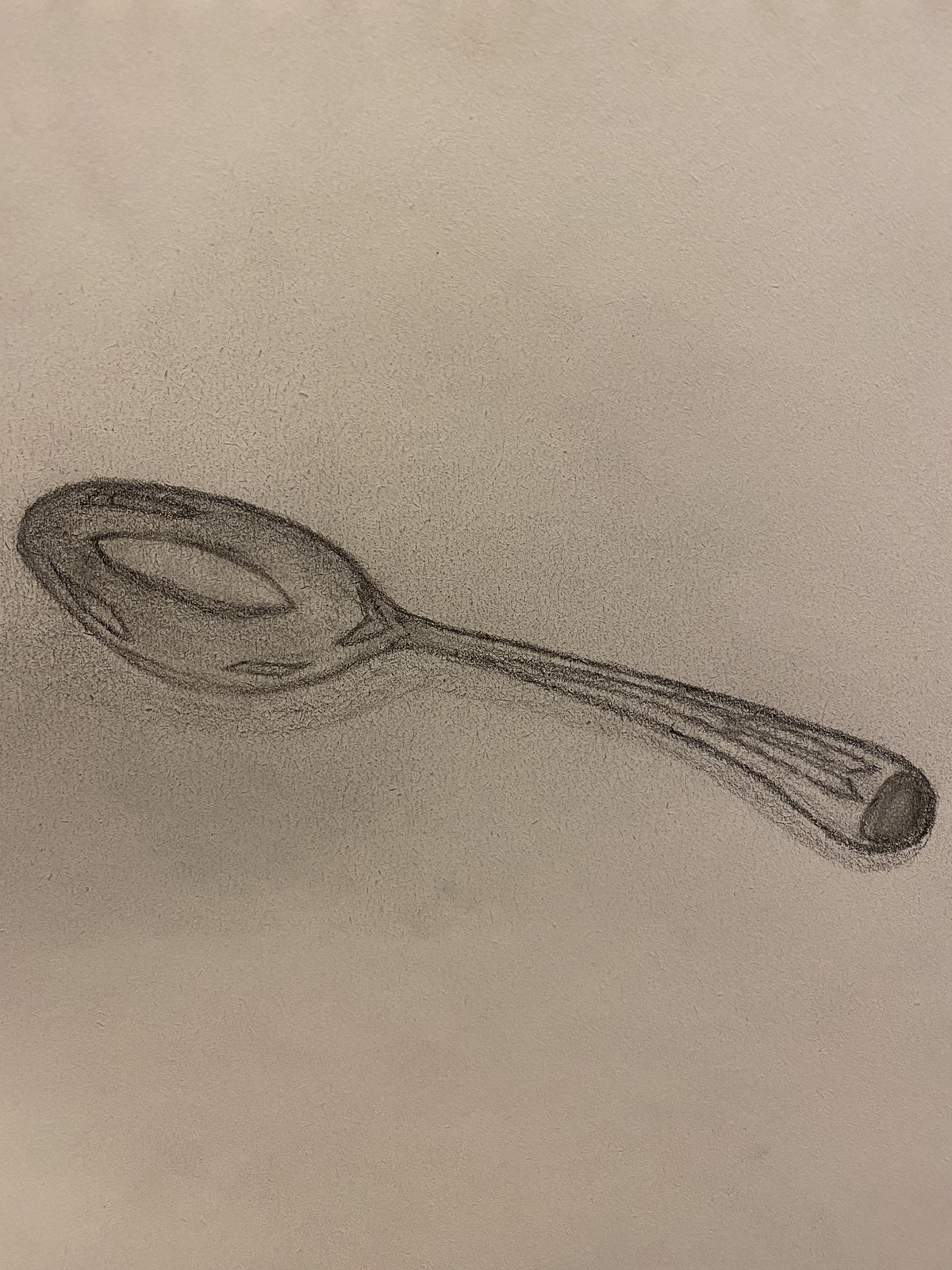This image features a detailed pencil drawing of a spoon on a white sheet of sketch paper. The spoon is centrally positioned, angled at approximately 40-50 degrees, with the rounded part on the left and the handle extending towards the lower right. The drawing employs a realistic graphite or charcoal style, with subtle shading beneath the spoon indicating a light source from above and slightly behind. The round bowl of the spoon features intricate shading, creating an effect of highlights and reflections, including a distinctive eye-like clear shape in the center. The handle showcases decorative lines resembling the arrows of a feather, leading to a black cap at the end. The background of the drawing remains plain white, emphasizing the solitary presence of the spoon.